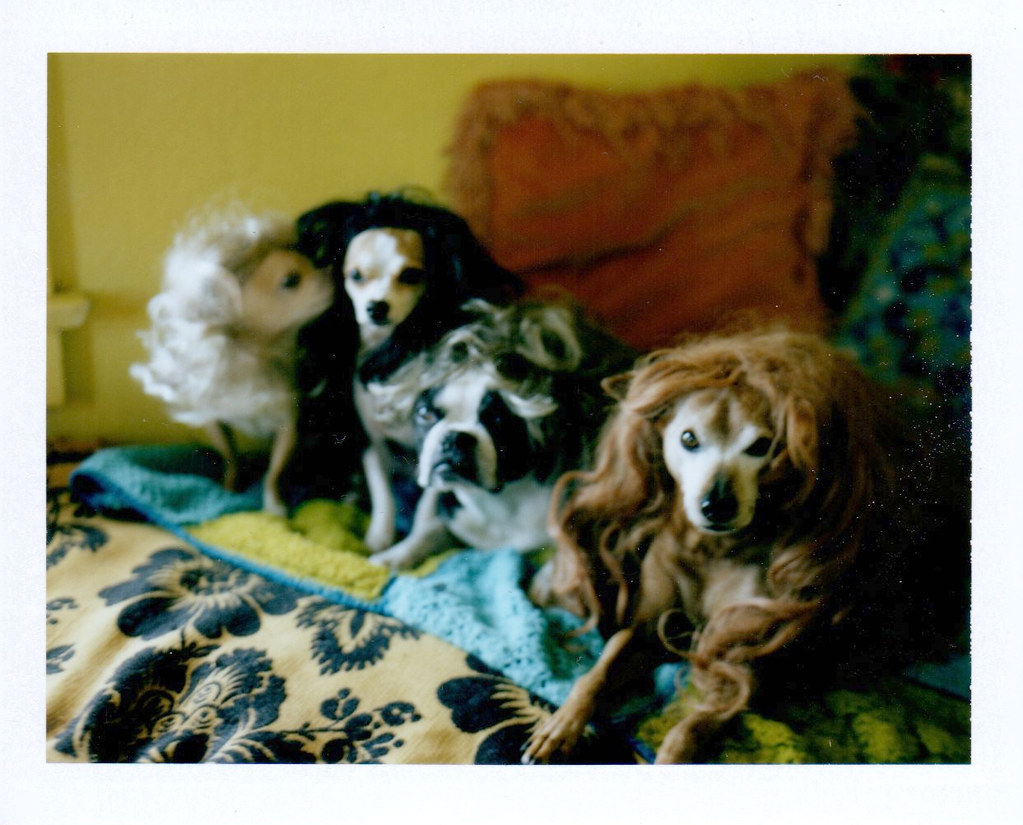The photograph depicts four dogs comfortably positioned on an indoor couch, flanked by throw pillows and covered with a blanket and a towel. Each dog is humorously adorned with an unkempt human wig that matches or contrasts its fur. From left to right: The first dog, a small brown chihuahua, wears a disheveled blonde wig and gazes towards the next dog. The second dog, another chihuahua with white and tan fur, sports a black wig. The third dog, slightly larger and chunkier with a white and tan coat, boasts a dark brown wig. Finally, the fourth dog, a light tan canine closest to the camera, is adorned with a brunette wig. Although the image, which appears somewhat old and worn with white specks of damage and a bit of a blur, shows varying focus across the dogs, it captures them all looking towards the camera, except for the leftmost chihuahua. Despite the degradation, the whimsical scene is clear: a cozy lineup of four small dogs, each playfully styled in a wig, set against the backdrop of a cream bedspread with black floral patterns.